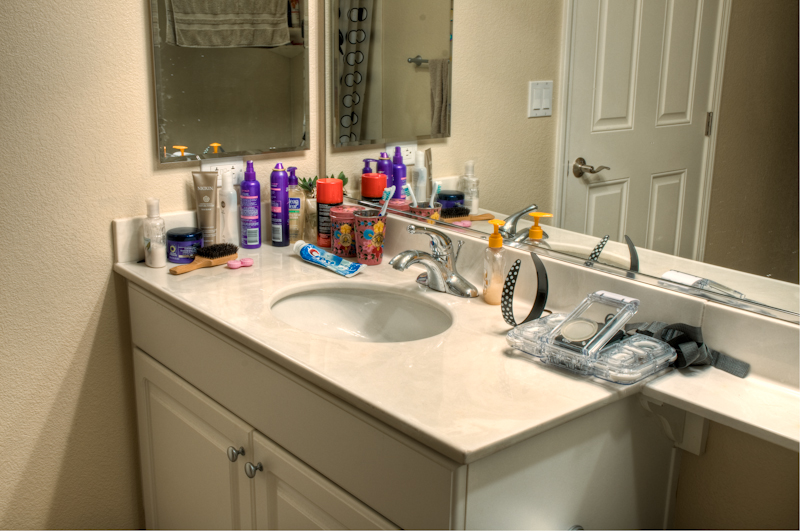In this rectangular photograph of a bathroom counter, the top and bottom sides are longer than the left and right sides. The left half of the image features a tan-painted wall, juxtaposed with a large mirror occupying the top one-fourth right section of the photograph. The mirror spans the entire length of the wall, reflecting everything in the room including the counter, a large white door set into a white frame with a silver-colored door handle, and a square light switch with two flat switches.

The countertop is tan-colored and features a large oval recess at its center, housing a white sink basin. Above the sink is a stainless steel, single-knob faucet. To the right of the faucet, there is a small clear plastic bottle filled with orange soap, topped with an orange pump-action dispenser. Further to the right, a black headband with white dots is standing on its flat, curved side.